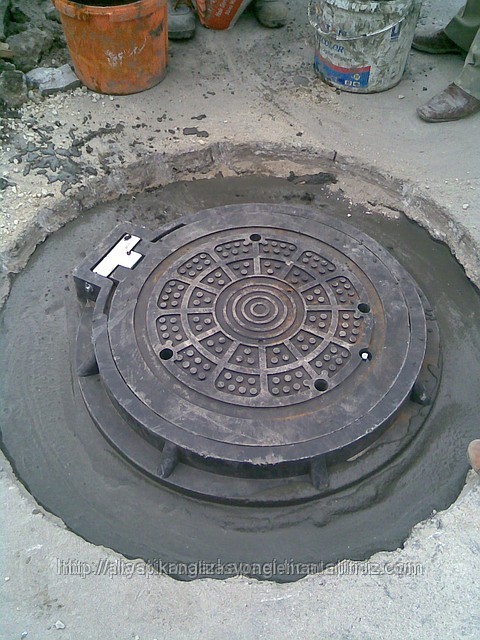The photograph, taken outdoors in daytime under medium light, focuses on a newly installed circular steel manhole cover set into a slightly larger circular opening. The manhole cover, which is a dark, iron-gray color with a detailed pattern of circles, lines, and dots divided into segments, contrasts with the fresh, still-wet concrete surrounding it. This freshly-poured concrete is roughly three to six inches below the level of the existing gray pavement, indicating ongoing work. 

In the foreground and background, the settled gray concrete surface shows some spillage and mess from the work. On the upper left, a dirty orange bucket is visible, while on the upper right, a five-gallon white bucket, also heavily soiled, likely used for mixing the concrete, sits adjacent to a workman’s shoes. A partially legible watermark of an undeciphered web address overlays the image, slightly blurred. The overall image is sharp and well-lit, capturing the unfinished state of the manhole cover installation and the surrounding construction materials.